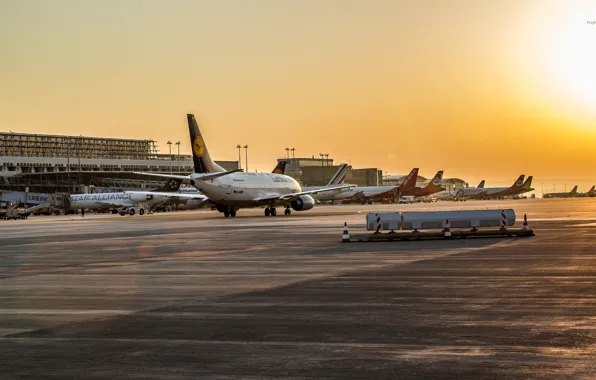The image captures a busy airport runway at sunset, with a large commercial airliner prominently featured in the center, gleaming under the sun's rays. The jet, with reddish wingtips, sits on a dark gray cement runway, ready for takeoff. To the left, multiple jets are parked near the airport terminal, which is outlined by various unlit lights atop its structure. The sky glows with a warm, yellowish-orange hue as the sun, appearing bright white in the top right corner, begins its descent, casting a golden light across the scene. On the right side of the image, cones and barriers are visible, ensuring proper navigation for the aircraft. The day appears to be partly cloudy, with the sunset's vibrant colors dominating the overcast sky. In the background, tall poles are faintly visible, completing the detailed landscape of this bustling airport environment.